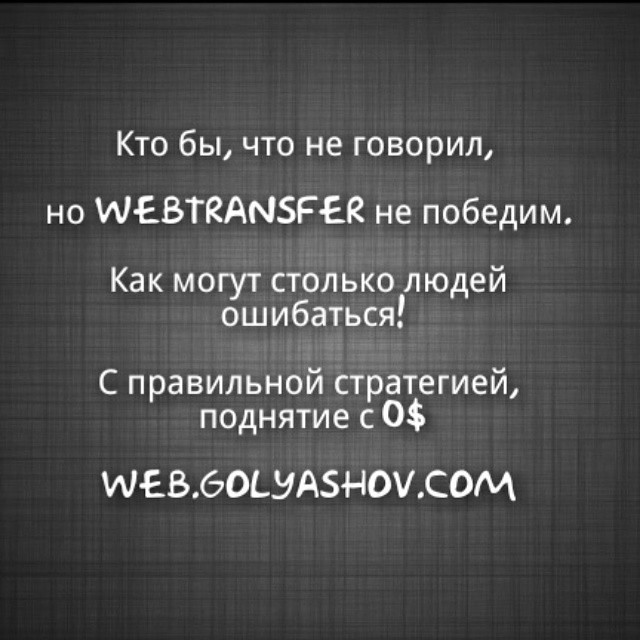The image features a textured black and gray background, upon which text is centrally positioned. The text is predominantly in Russian, but certain elements stand out in English, such as "web transfer" prominently displayed in capital letters. Additional noticeable components include a string of Russian words and characters, and at the bottom of the image, a web address: "web.golyashov.com." Above the web address, there are symbols like a zero, a dollar sign, and an 'S' with a vertical line through it. The background exhibits a gradient from dark to light gray with dark vertical lines, enhancing the stitched appearance. Overall, the image appears to be an advertisement for a website, characterized by its monochromatic color scheme of blacks, grays, and whites.